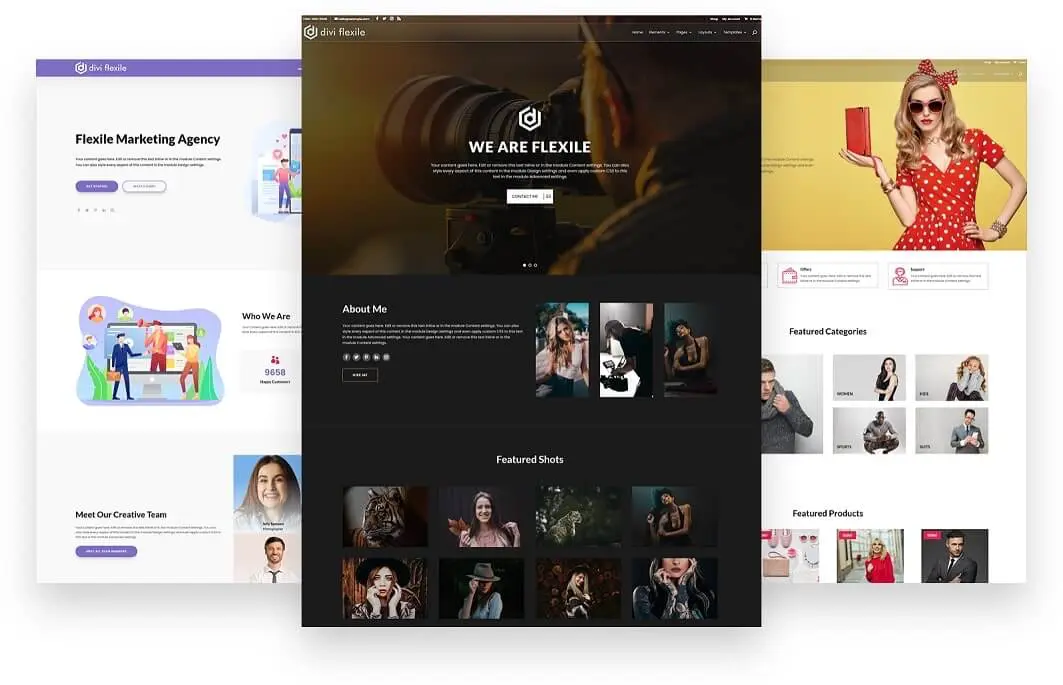The image features a tri-screen layout, divided into three distinct sections.

**Center Panel:**
In the middle panel, a dominant dark red background is topped with white text. On the right side of this panel, there's a list numbered from 1 to 6, although the text is too small to be legible. A peculiar logo is displayed here, and in the background, an individual – partially obscured and bathed in an orangish-red tint – appears to be drinking from a water bottle, which is actually revealed to be a large digital camera upon closer inspection. The text "We are flexible" is prominently displayed, accompanied by an overwhelming amount of white text underneath it that is essentially unreadable. A notable white button is also present.

**Left Panel:**
On the left side of the tri-screen, the background is primarily black with white text at the top reading "About Me". This section contains a wealth of information and various images, likely representing this person’s work or hobbies. A specific image towards the top features a blue line with white text against a white background and black text detailing "Flexible Marketing Agency". The panel includes black, blue, and white buttons for interaction, mirroring some elements from the center panel.

**Right Panel:**
The rightmost section of the image features a photograph of a woman looking directly at the camera. She is dressed in a red sundress and black sunglasses, her hair is styled in a bun, and she holds an unidentified red object in her left hand. Her pose conveys a confident "look at me, I'm cool" vibe. Below her, there are additional images which appear to be generic stock photos.

Overall, the tri-screen seems to be showcasing a blend of personal branding, marketing content, and interactive elements, although much of the detailed text remains unreadable.